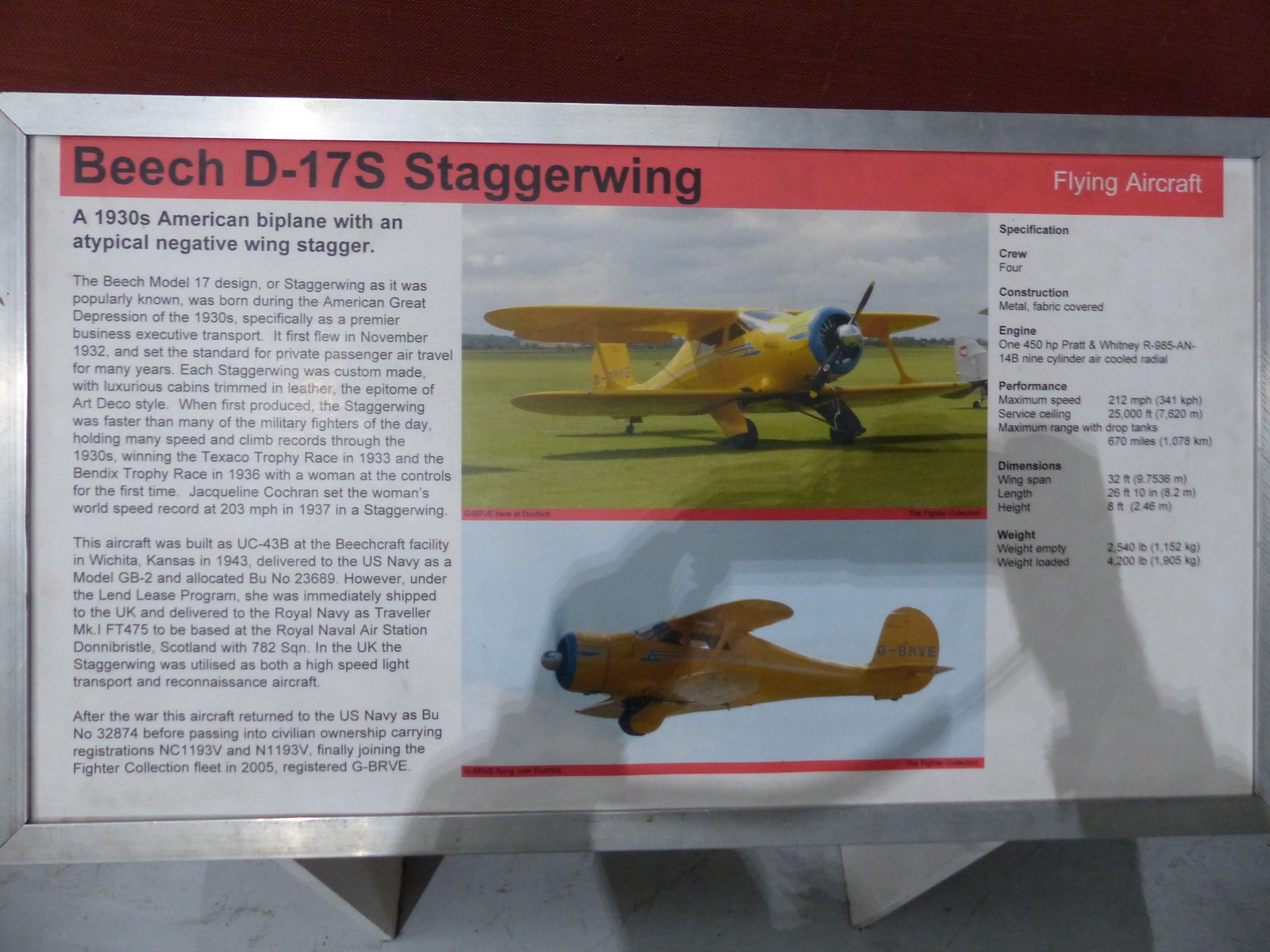This detailed image depicts an informational poster about the Beach D-17 Stagger Wing, a 1930s American biplane characterized by an atypical negative wing stagger. The poster features a prominent red bar across the top with black text that states "Beach D-17 Stagger Wing" and additional white text that reads "Flying Aircraft." Two photographs of the yellow aircraft are included: one of it resting on the ground in a grassy area and the other capturing it mid-flight. Notably, the plane has a blue tip on the nose, just before the propellers. 

On the left-hand side, there's a description that reads, "1930s American biplane with an atypical negative wing stagger." The right-hand side lists detailed specifications, including:
- **Crew:** 4
- **Construction:** Metal fabric-covered
- **Engine:** 1 x 450 HP Pratt & Whitney R985 AN-14B 9-cylinder air-cooled radial
- **Performance:**
  - Maximum Speed: 212 miles per hour (341 kilometers per hour)
  - Service Ceiling: 25,000 feet (7,620 meters)
  - Maximum Range with Drop Tank: 670 miles (1,078 kilometers)
- **Dimensions:**
  - Wingspan: 32 feet (9.75 meters)
  - Length: 26 feet 10 inches (8.2 meters)
  - Height: 8 feet (2.46 meters)
- **Weight:**
  - Empty: 2,540 pounds (1,152 kilograms)
  - Loaded: 4,200 pounds (1,905 kilograms)

This placard is likely found at an air show or an aviation museum.